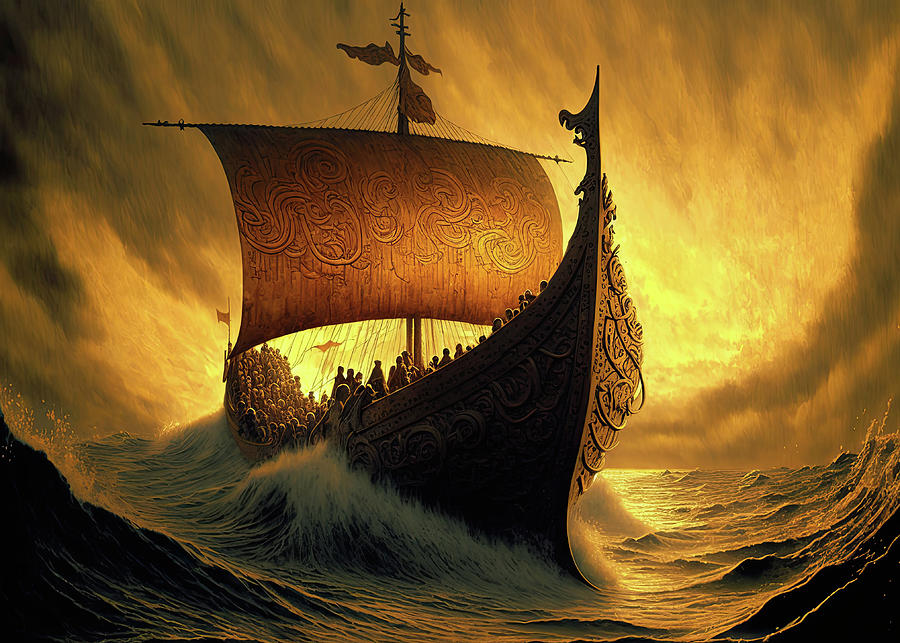The image is a horizontally aligned rectangular painting depicting a dramatic and tempestuous maritime scene. The background showcases a tumultuous sky filled with swirling clouds that transition from dark browns at the top to golden yellows towards the bottom, giving the sky a glowing, almost ethereal quality. A large, antique ship, reminiscent of a Viking vessel, dominates the foreground. The ship features a prominently curved and sharply pointed front and an intricate crown molding along its sides, akin to ornate leaf patterns. A massive rectangular sail, adorned with similar wavy, curvy leaf designs, rises from the center of the ship. The interior of the ship is densely packed with people, all huddled closely together. Surrounding the vessel, large, powerful waves with bluish-gray hues and frothy white caps crash against its sides, especially prominent on the left and right corners of the image. The overall scene conveys a sense of peril and grandeur as the ship battles the formidable, wavy sea beneath the ominous yet glowing sky.